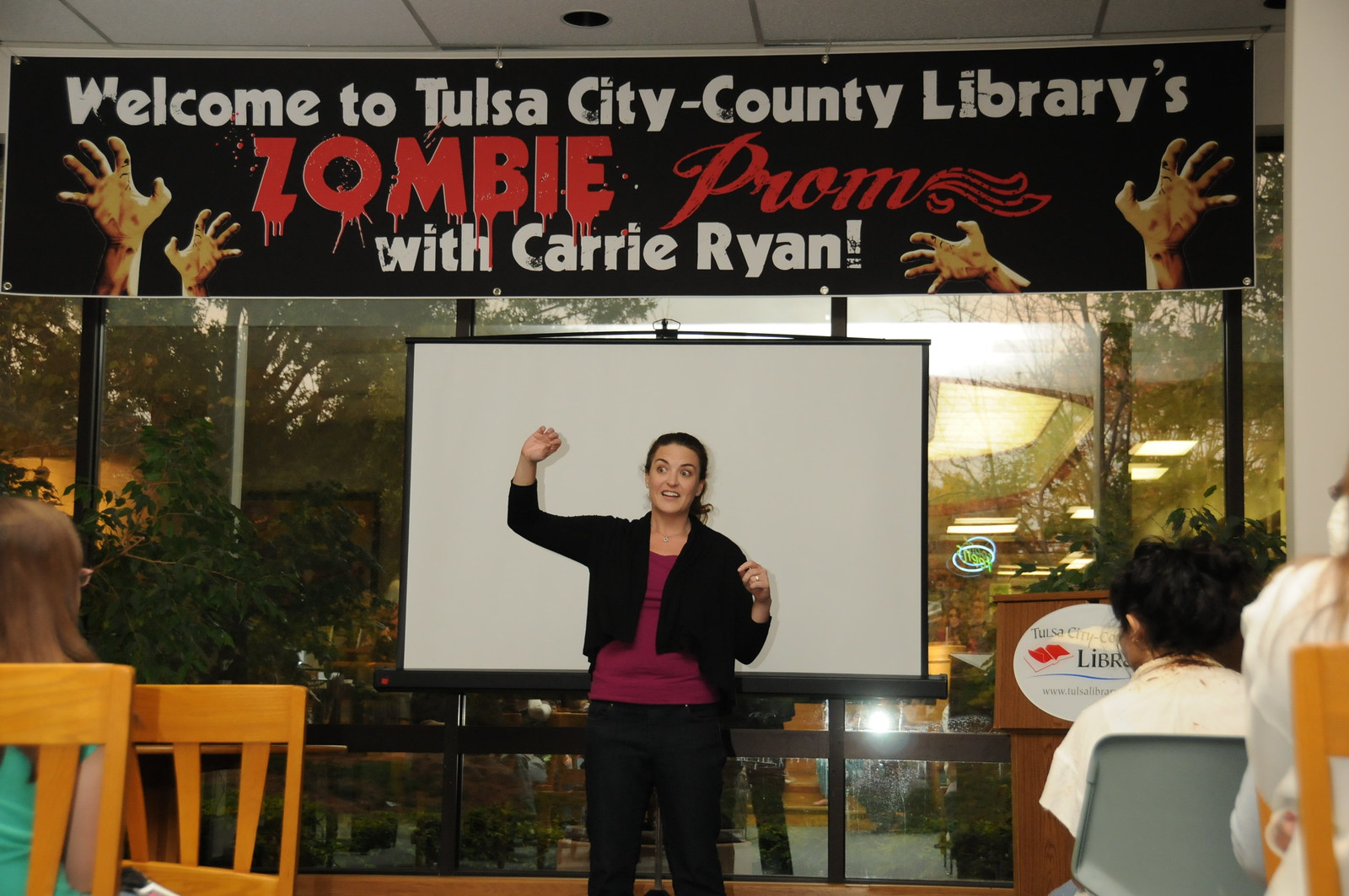In this indoor photograph, we see a woman giving a presentation at the Tulsa City-County Libraries. She stands in front of a silver video projector screen, wearing a black jacket over a magenta shirt, and black pants. Her black hair frames her face as she raises her right arm up, gesturing towards her audience. Above her, a banner stretches across the top of the image, reading "Welcome to Tulsa City-County Libraries Zombie Prom with Carrie Ryan." The word "Zombie" is displayed in a bloody, dripping red horror-movie font, while "Prom" is also in red but without the dripping effect. Decorative green zombie hands are visible in the bottom corners of the banner. The audience, consisting of children sitting on gray and wooden golden chairs, listens attentively. Behind them, windows and indoor plants are visible, confirming the photograph was taken indoors.